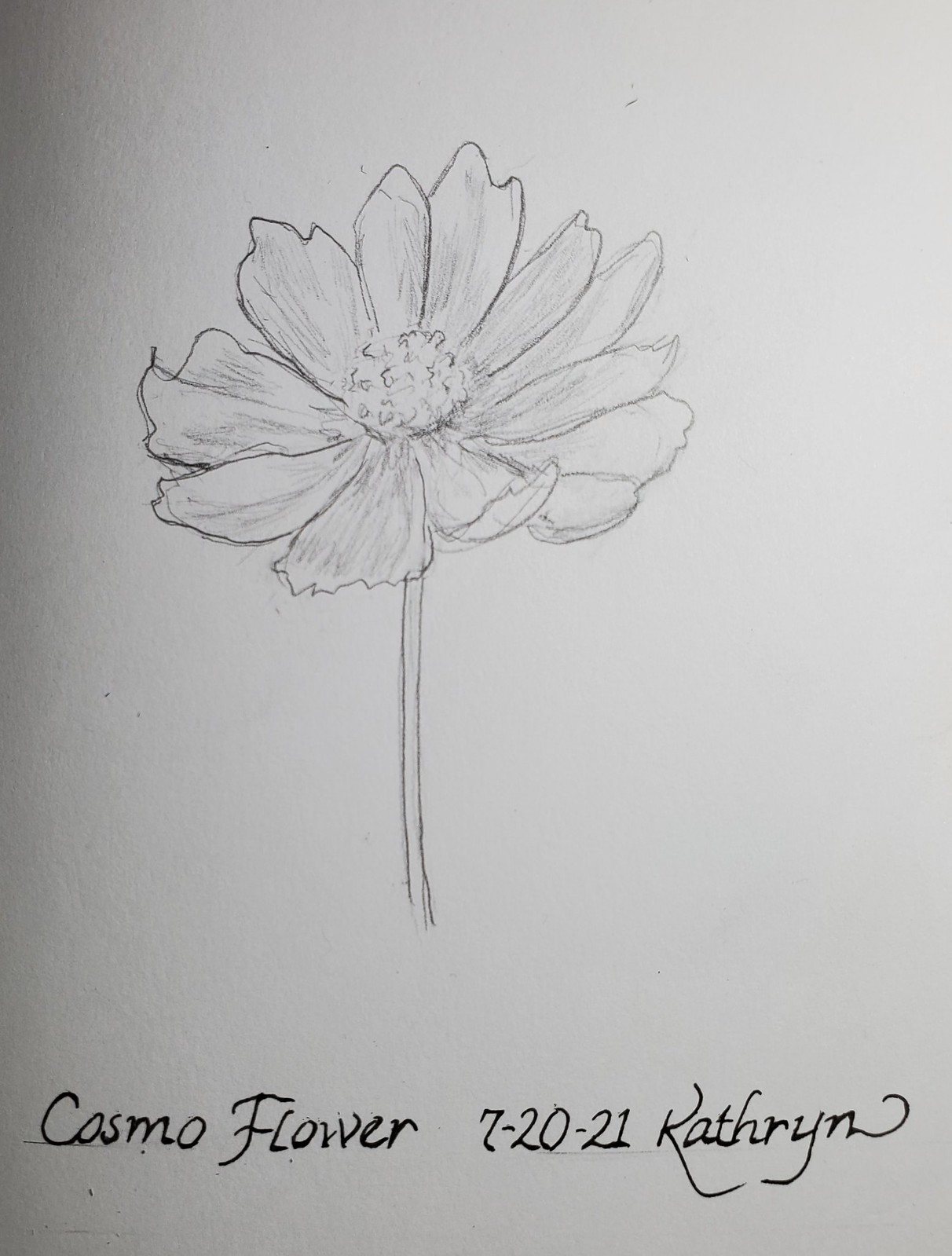This detailed caption has been crafted for an image of an artwork:

---

A meticulously hand-drawn illustration of a fully blossomed flower titled "Cosmo Flower" is presented at the bottom of the page. The artist, Catherine, has carefully aligned the title, date, and her signature horizontally across the top, employing a faint guideline that has been partially erased, but its remnant still visible. The piece is dated July 20th, 2021. The flower, featuring around 14 to 15 delicate petals, reveals a densely textured central area, reminiscent of abundant pollen. A simple, minimalist stem completes the elegant botanical sketch. Rendered in pencil with subtle accents of pen, the artwork displays a monochromatic palette of blacks and grays, devoid of any color.